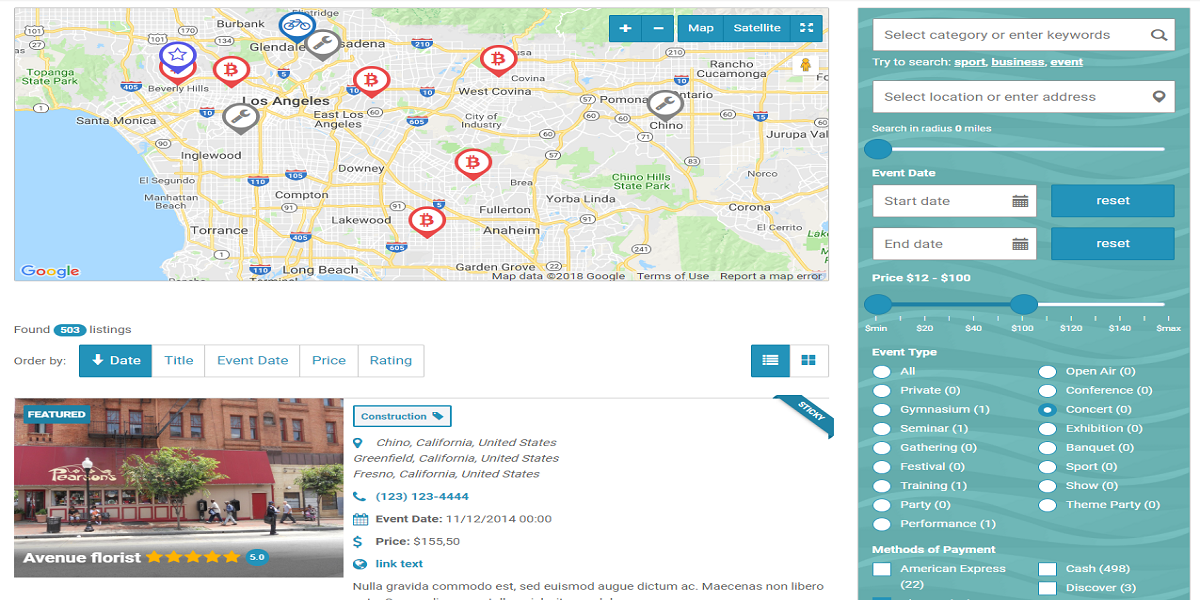The image features a detailed event search interface with a map of Los Angeles prominently displayed on the left side. The right side of the screen is occupied by a comprehensive search menu set against a dark green background. The menu is divided into several input fields: 

1. **First Field:** Prompts users to either select from the category "Kazakori" or enter keywords such as "sports," "business," and "events."
2. **Second Field:** Allows users to select a location or enter a specific address. Additionally, there is a configurable radius slider for search results, measured in miles.
3. **Event Date Section:** Includes input fields for both a start and end date, with options to pick specific dates from calendar pop-ups.
4. **Price Range Slider:** Enables users to set a minimum and maximum price range for events.
5. **Event Type Selection:** Users can filter events by type, including options such as "All," "Private," "Gymnasium," "Seminar," "Gathering," "Festival," "Training," "Party," "Performance," "Open Air," "Conference," "Concert," "Exhibition," "Banquet," "Sports," "Show," and "Theme Park." In this instance, "Concert" is selected.
6. **Payment Methods:** The bottom of the menu features checkboxes for payment methods: American Express, Cash, or Discount.

Below the map, a summary section shows:
- **Search Results:** "Found 503 listings."
- **Sorting Options:** Users can sort results by date, title, event date, pricing, or rating.

A highlighted event features:
- **Event Name:** Avenue Florist
- **Rating:** 5 stars
- **Locations:** Chino, California, United States; Greenfield, California; Fresno, United States
- **Contact Number:** 123-123-4444
- **Event Date and Time:** November 12th, 14:00 (2:00 PM)
- **Price:** $155.50
- **Link Text and Button:** Displayed in blue.

Overall, the interface is user-friendly and allows for detailed, customizable event searches within the Los Angeles area.